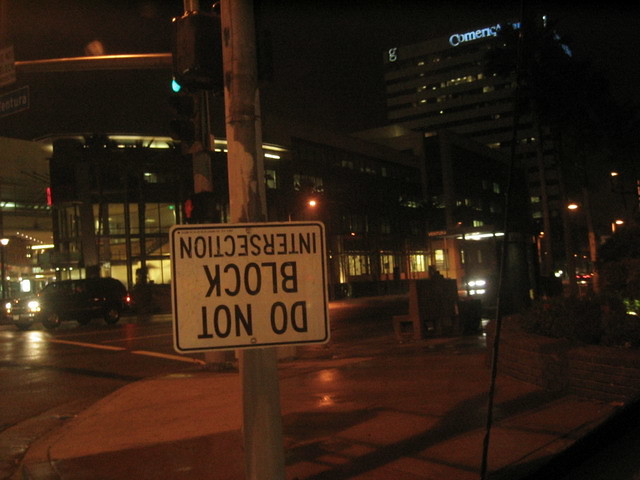This detailed night-time photograph captures a busy urban intersection. At the right side of the frame, an SUV with its headlights on waits at a red light. Central to the image is a metal pole with a sign that reads "Do not block intersection," but the sign has fallen and is now upside down. To the left of center, another vehicle is captured in motion, moving from right to left. Beyond the intersection, various buildings line the background. A high-rise hotel displaying the word "OMENS" in illuminated letters stands out among the structures, with many of its rooms lit up. A tall white building also features prominently, bearing partial signage that reads "Comen" as its left side is obscured by a large, dark palm tree. Additional details include a glass building, a parking garage, and a nearby bus stop complete with a bench. The sky above is dark, lacking visible stars or the moon, adding to the scene’s nocturnal atmosphere.